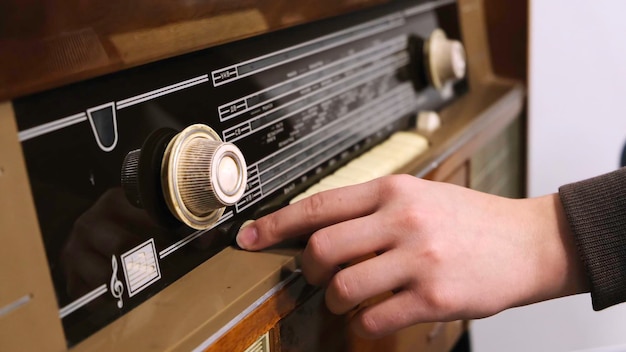The image showcases an old, nostalgia-inducing piece of musical electronic equipment that appears to be a radio from the 1950s. The radio is encased in a combination of brown plastic and wood, exuding a vintage aesthetic. It features a black front panel adorned with two white, slightly dirty dials, likely used for tuning radio frequencies or stations. Beneath each dial are white buttons, possibly serving as presets. Additionally, a musical clef symbol is prominently displayed on the bottom left of the radio, reinforcing its musical functionality. In the foreground, a hand clad in a long-sleeved sweatshirt enters from the right side of the frame, with the index finger extended towards the closest dial, suggesting an intent to adjust the settings. The overall scene is captured within a cabinet, adding to the retro atmosphere of the image.